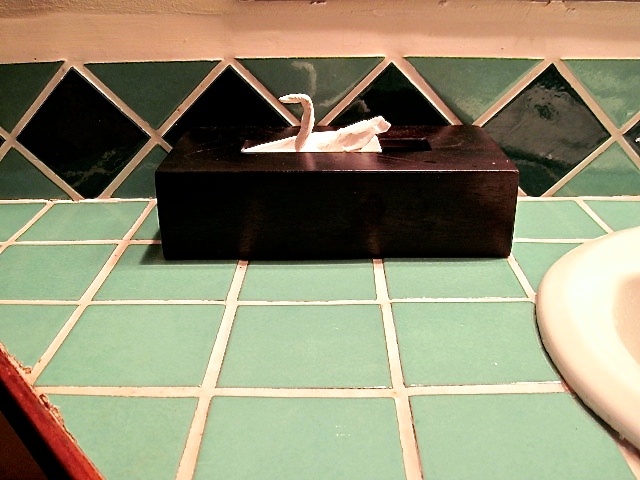This detailed photograph showcases an extreme close-up of a bathroom counter featuring green tiles. At the center of the image, a black tissue box stands prominently, with a tissue artistically folded into the shape of a swan emerging from the box. The backsplash behind the tissue box consists of a stripe design made up of green and black tiles, with black tiles arranged in a diamond pattern within the green stripe. To the far right, the ceramic or porcelain rim of a sink basin is visible. The lower right corner reveals the end of the counter leading to a dark area, presumably the floor or space beneath the counter. The scene is well-lit, emphasizing the details, including the lower left corner where the edge of the counter shows noticeable wear and tear. The tiles appear cracked and have been repaired with caulk, reflecting the counter's aged and used condition.